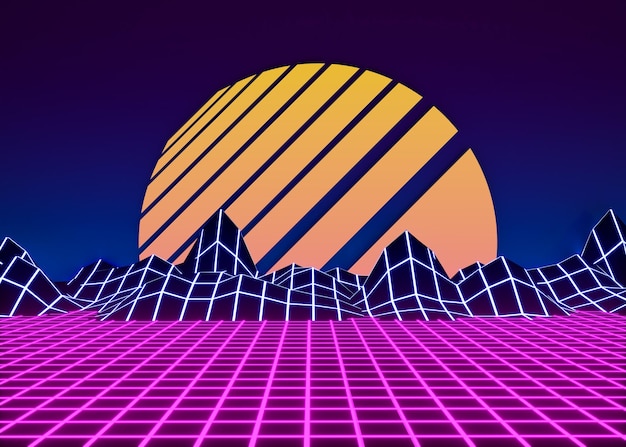The image is a vibrant and animated scene dominated by bright and bold colors. At the bottom is a vivid neon purple grid, forming small squares as though representing land or terrain. This purple grid transitions into a jagged, mountainous area depicted in dark purple and black, overlaid with neon blue lines that intersect to create varying sizes of squares. Rising above these mountains is a large, semi-circle sun, which spans from the right to the left side of the image. The sun is a striking yellow that fades to orange, and it is bisected by thick diagonal blue lines that taper from wider on the right to thinner on the left. The entire scene is set against a deep royal blue background that transitions from lighter near the sun to a darker blue towards the top of the picture. The overall design appears computer-generated, with a clear structure and a vivid, neon aesthetic that makes the image strikingly bright and dynamic.